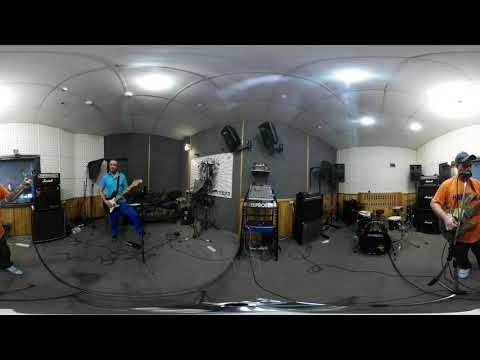This detailed indoor scene captures a bustling recording studio filled with musical instruments and equipment. Dominating the left side of the image, a man in a blue shirt and dark blue pants holds an electric guitar, poised for a session. To his right, another man stands wearing a blue ball cap, an orange t-shirt, pants, and white sneakers, also clutching an electric guitar. Both men appear to be Caucasian. The space is densely populated with various audio equipment and speakers, arranged along the grayish floor and mounted on the white and partially carpeted walls. Overhead, six ceiling-mounted lights illuminate the room. In the background, a drum set awaits use, accompanied by black file cabinets and an array of wires crisscrossing the floor. A hint of a window on the far left suggests a possible adjacent room. The setting conveys a dynamic and well-equipped environment, ready for a recording session.